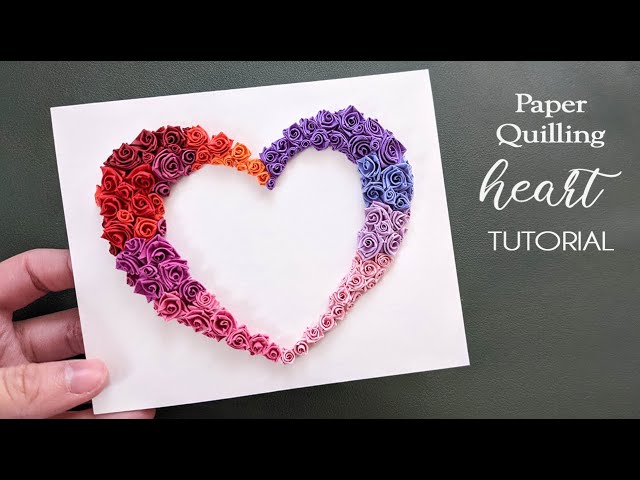The promotional image showcases a detailed header banner for a tutorial on creating a paper quilled heart. The image features solid black borders along the top and bottom, framing the central photograph. On the right side, white text reads, "Paper Quilling Heart Tutorial." On the left, a light-colored human hand holds a small rectangular piece of white cardstock adorned with a meticulously crafted heart. This heart consists of various handmade paper rosettes arranged in a beautiful ombre pattern: pink rosettes start at the bottom right transitioning through purple, blue, and dark purple at the top; the bottom left showcases dark purple blending into lilac, red, dark red, and orange. The hand holding the card is unadorned, without nail polish. Beneath the hand's position, there is a textured black surface, likely a table. This image serves as an enticing visual guide, possibly as a thumbnail for a comprehensive video tutorial, instructing viewers on how to create this intricate and visually appealing craft.